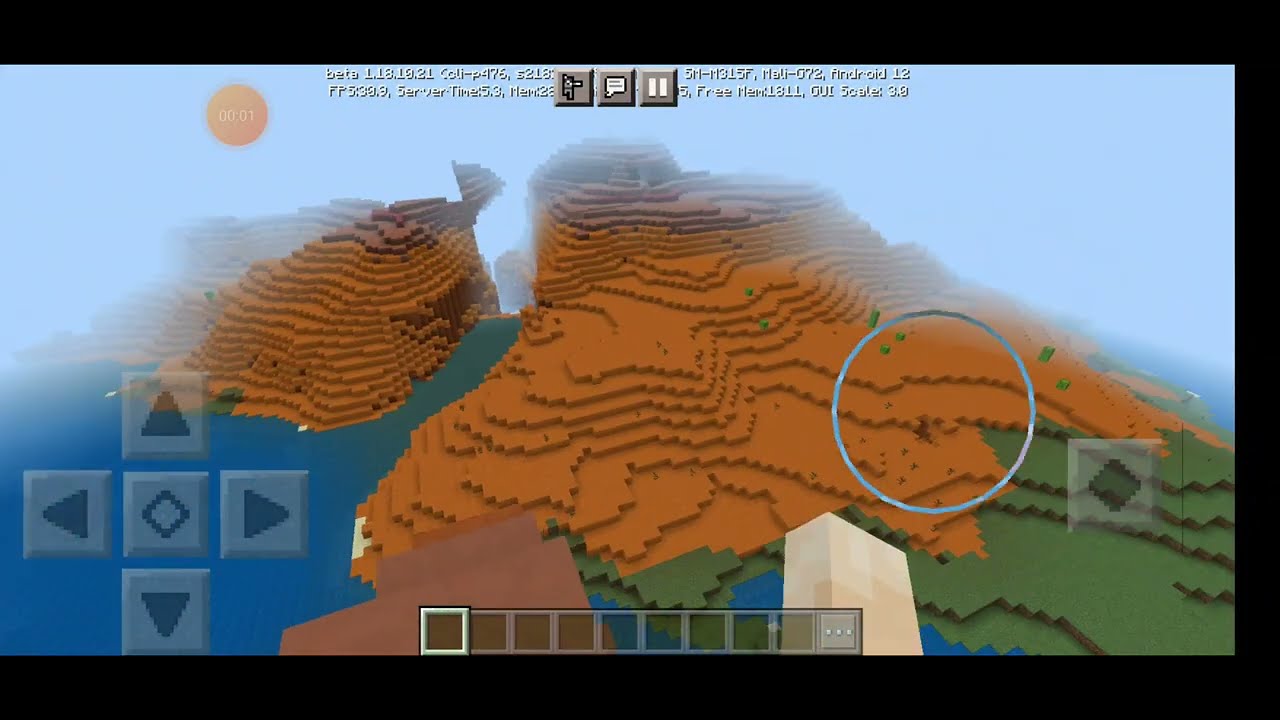The image is a screen capture from a pixelated, Minecraft-like video game with a prominent 8-bit graphical style. The game view is aerial, looking down at a divided landmass. The bottom left features a flat expanse of blue water, presumably a body of water, which runs through the center as a river, separating two mountainous regions. The mountains have green bases that transition to light brown and then to dark brown peaks. The screen itself is bordered in black, with a thinner border on the right side. At the top of the screen, there are three buttons from left to right: an indiscernible icon, a speech bubble, and a pause symbol. The top also shows an indistinct text area, possibly for game information or narration. The bottom part of the screen includes a directional pad with arrows for movement in the bottom left and a series of nondescript button icons or actions stretching across the bottom. The visual composition resembles a topographical map with detailed terrain features.